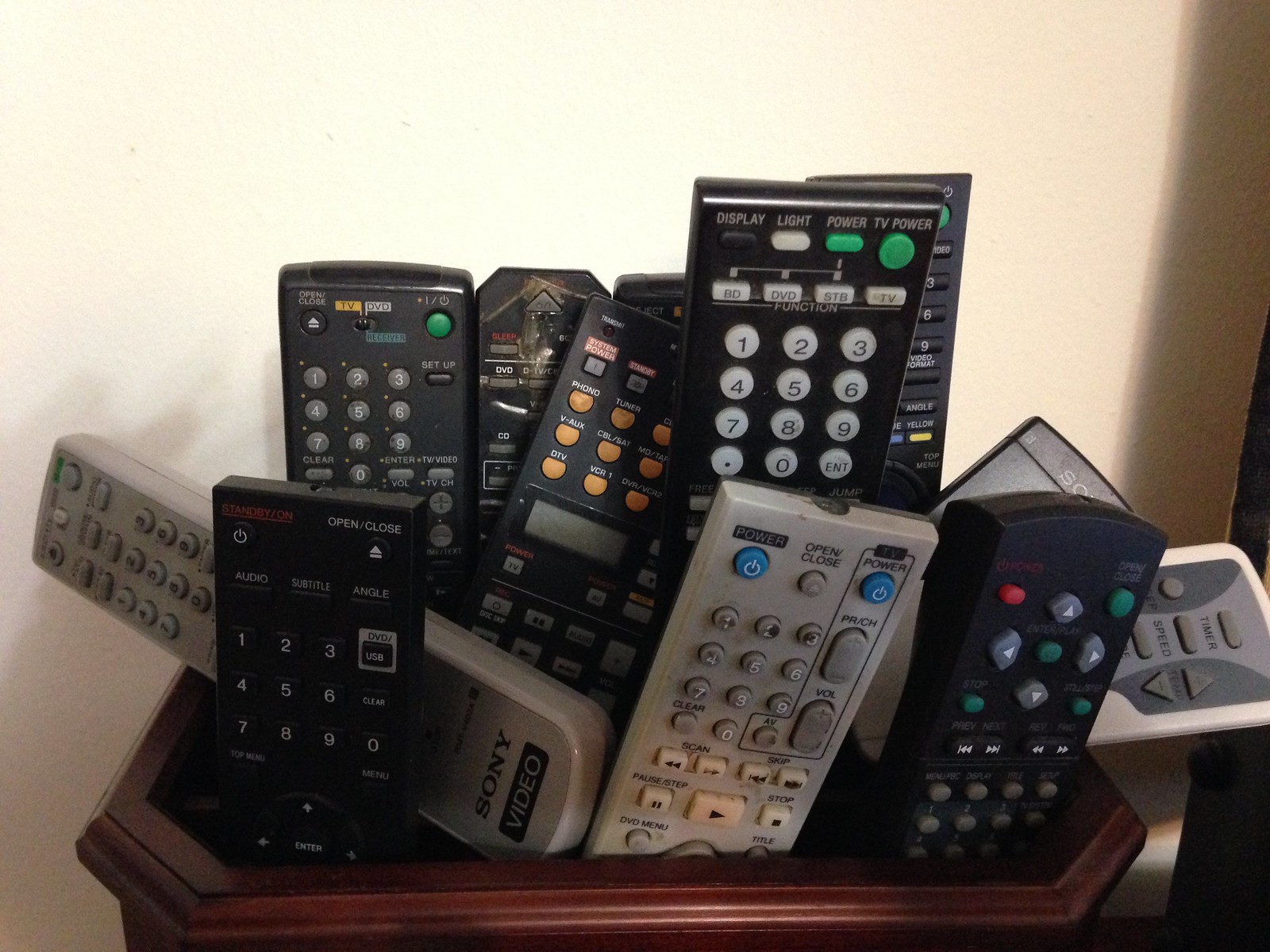The photograph displays a low-light indoor scene centered on a small, dark wooden container filled with a variety of remote controls. The container, which has an elongated diamond shape, sits against a white wall with a slight yellow tint on the right side. Inside the container, there are twelve remote controls, arranged in a somewhat orderly manner but some are leaning or tipped over. 

Among the remotes, nine are black and three are a light gray or beigy white color. The remotes are different brands, with one prominently displaying "Sony Video" at the bottom. The buttons on the remotes vary in color, including green, yellow, blue, orange, and white, indicating they are for various functions. The remotes have different shapes, mostly rectangular, with some being more oblong and blocky.

Overall, the image captures a scene of used remote controls stored in a cherry wood-like container, showing signs of wear and various colored buttons, under low-light conditions with a white wall in the background.